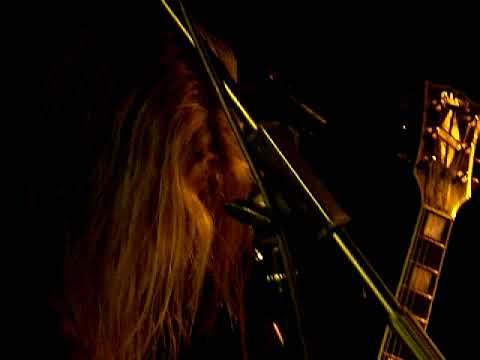The image depicts a close-up scene that appears to be taken from a video of a musical performance. In the foreground, the top half of a black and gold electric guitar is visible on the far right side, its silver strings catching the light. The head of a microphone stand occupies the center of the frame, leading up to a mass of long blonde hair that suggests the musician's head is either bowed or covered while performing. Details of the musician’s face are obscured by the hair, hinting at a dynamic moment such as headbanging. The background is pitch black, intensifying the focus on the few illuminated elements: the guitar, the hair, and the microphone stand. The aesthetic suggests a dimly lit, intimate stage setup often found in live musical performances.